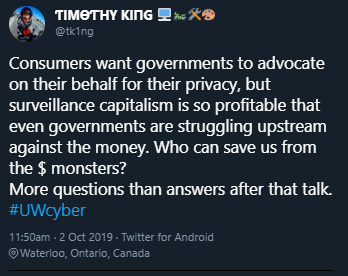The image features a square frame with a black background. At the top of the image, there is a circular profile picture of a person against a blue sky background. The person is wearing a combat helmet. Below the profile picture, the user's name, "Timothy King," is displayed, accompanied by icons depicting a computer screen, tools, and an art easel or palette.

Below the name, the text "@TK1NG" is prominently shown. The post content is written in white text and states: "Consumers want governments to advocate on their behalf for their privacy, but surveillance capitalism is so profitable that even governments are struggling upstream against the money. Who can save us from the dollar monsters?" followed by a dollar sign graphic.

At the bottom, the phrase "More questions than answers after that talk" is visible, and in blue text, the hashtag "#UWCYBER" is included.